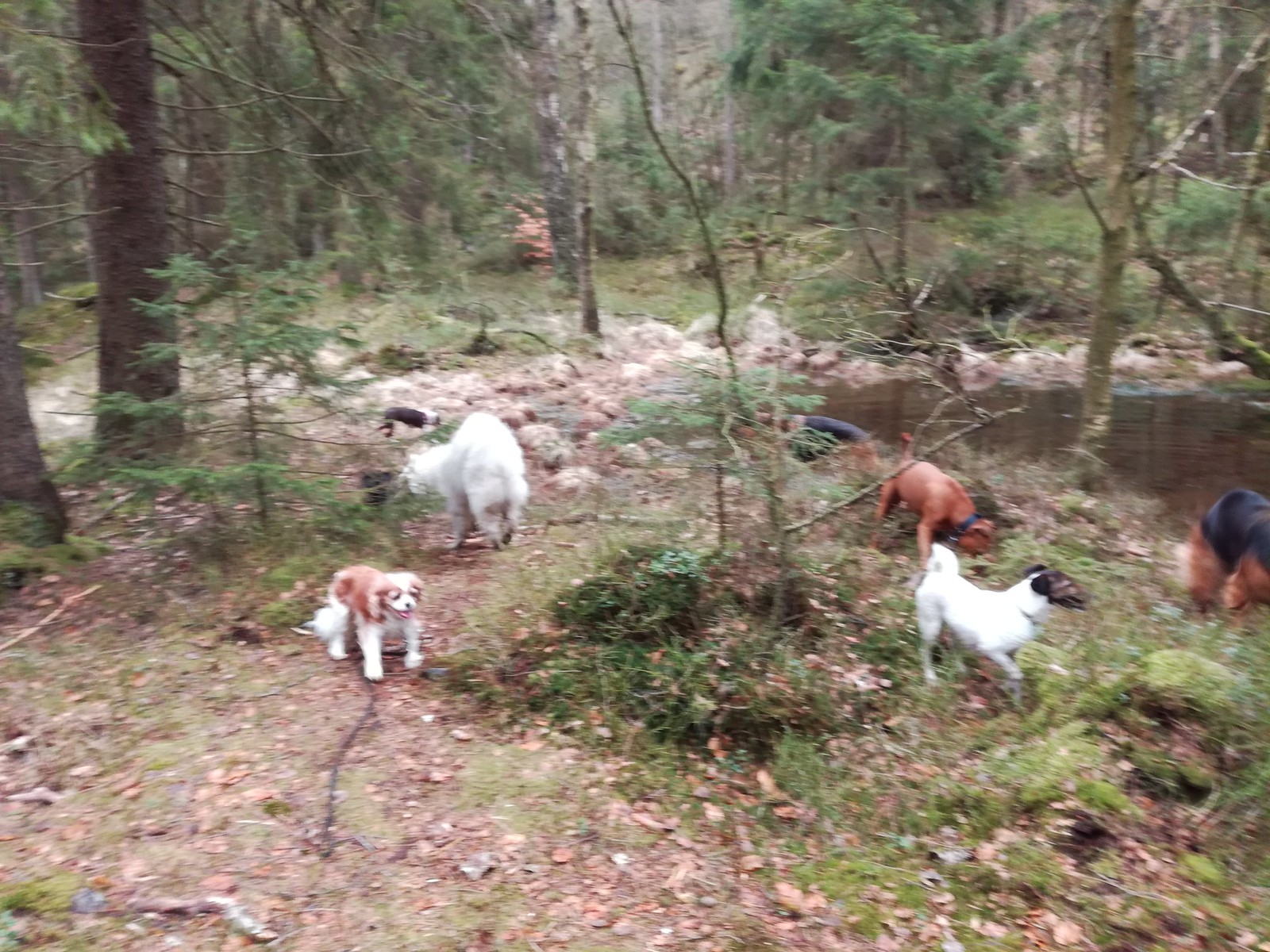This detailed photograph captures a vibrant outdoor scene, likely taken during a sunny late summer or early fall day in the woods. The setting features a variety of green trees, bushes, and pine trees, with a hard, dried mud floor scattered with leaves, twigs, rocks, and light brown bushes. Towards the right side of the image, there is a small, brownish creek or pond, surrounded by additional greenery.

In the foreground and background, a group of five to six dogs of various breeds and colors are energetically exploring the area, without leashes. There's a Jack Russell Terrier, a Cocker Spaniel, and a Beagle among them. The dogs display a range of color patterns: there are three white dogs—one large, one small with a black head, and another small with rust-colored fur on its back and head. There is also a rust-colored dog with a dark collar sniffing the ground, and another rust-colored dog with black fur on its back. In the distant background, there may be another small dog, primarily black with a white head, though it is difficult to discern clearly. The overall lively atmosphere suggests that the dogs are either hunting or simply frolicking around and enjoying their time in nature. One of the dog's owners might be capturing this picturesque moment.